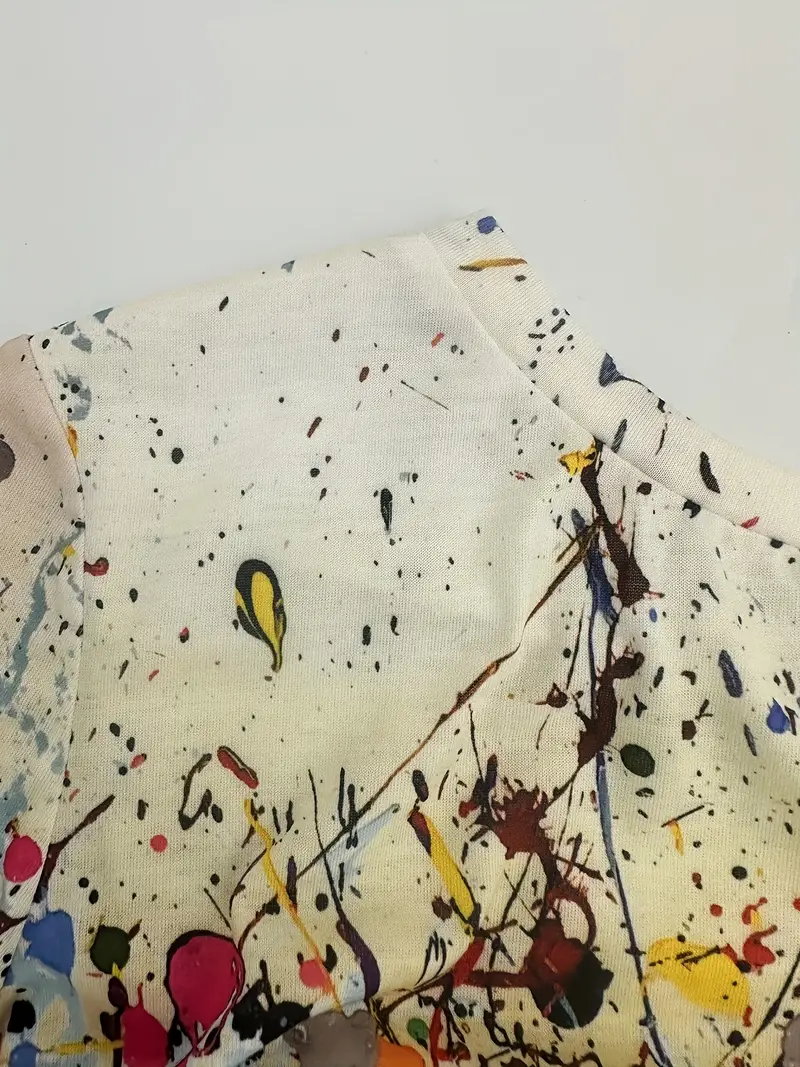The image features a white t-shirt with a modern abstract art design. The shirt lies on a white surface, displaying just the neck, right shoulder, and a touch of the sleeve. The fabric is adorned with a chaotic array of multicolored paint splatters, reminiscent of a Jackson Pollock painting. The splatters include blues, blacks, greens, reds, purples, yellows, and browns, applied in random patterns without specific order. Notable details include clusters of little black spots, large red splotches at the bottom left, brown streaks running diagonally from the bottom left to top right, and gray streaks moving vertically. This meticulous combination of vibrant colors against the plain white background creates a striking and dynamic piece of wearable art.